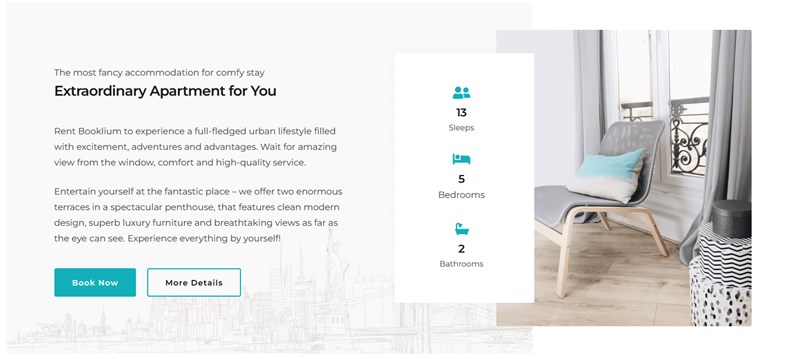This image captures a webpage advertising an upscale apartment. The primary text at the top reads, "The most fancy combination for your company's stay: coffee stay." Below this in prominent, bold letters is the phrase, "Extraordinary Art Apartment for You." On the right side of the image, a rectangular section contains icons and text: a people icon followed by "13 sleeps," a bed icon with "5 bedrooms," and a tub icon indicating "2 bathrooms." To the left, there is a picture of an elegant pillow on a stylish chair. 

To the right of this image, additional promotional text invites readers to "Rent Book Liam" to experience a comprehensive urban lifestyle filled with excitement, adventure, and advantages. The description promises an amazing view from the window, comfort, high-quality service, and the opportunity to rejuvenate in a fantastic setting.